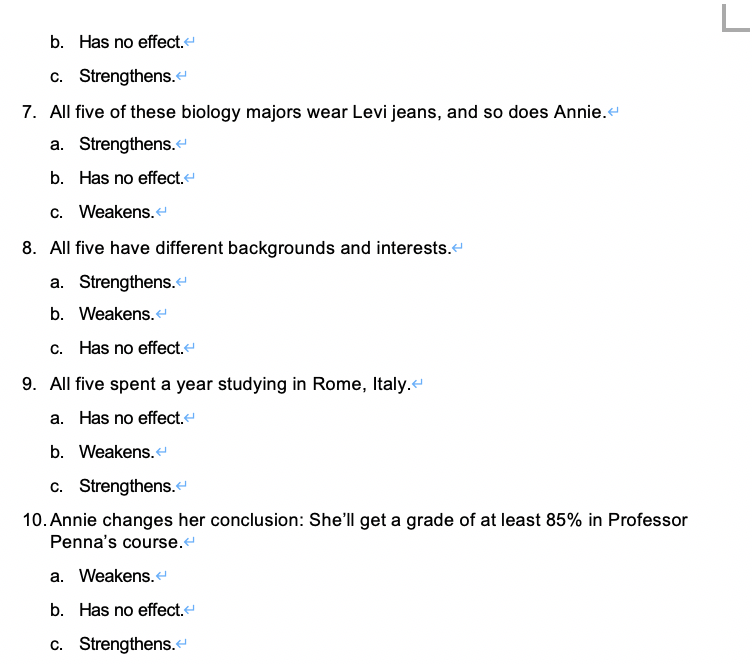This image features a multiple-choice question set against a white background with black text. Each question from 7 to 10 is associated with options A, B, and C. The number 6 is partially obscured, but options B and C for number 6 are visible. At the end of each line of text, there is a blue arrow indicating a specific direction, referred to as an "anti-arrow."

- For number 6, the text states: "B has no effect, C strengthens."
- For number 7, it mentions: "All five of these biology majors were left by Jean and so does Annie. A strengthens, B has no effect, C weakens."
- For number 8, it remarks: "All five have different backgrounds and interests. A strengthens, B weakens, C has no effect."
- For number 9, it declares: "All five spent a year studying in Rome, Italy. A has no effect, B weakens, C strengthens."
- For number 10, it concludes: "Annie changes her conclusion. She will get a grade of at least 85% in Professor Penna's course. A weakens, B has no effect, C strengthens."

Participants are instructed to select A, B, or C based on whether the option strengthens, weakens, or has no effect in the context provided.